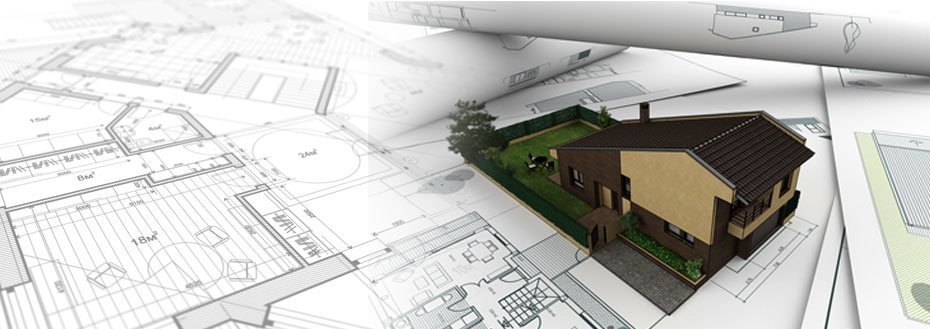The image features detailed architectural drawings and a 3D model of a house. The blueprints, showcasing the layout of various rooms including bathrooms, dining rooms, bedrooms, and the kitchen, are predominantly rendered in white, gray, and black ink. These floor plans are laid out diagonally, with one rolled-up blueprint positioned at the top right of the image. Centered within the photo lies a sophisticated computerized model of a house, characterized by its brown and tan khaki walls and unique roof design, with the chimney notably placed on the left. This model sits atop the blueprints, representing the interior layout of the house. The house includes an L-shaped backyard, featuring a tree in the top left corner and a green fence, offering a realistic touch to the presentation.